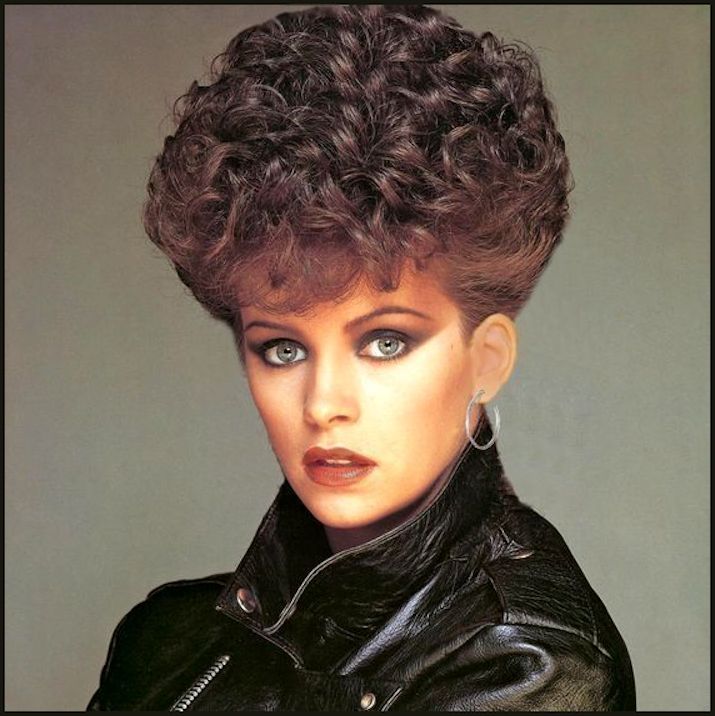This portrait features singer Sheena Easton set against a light gray background. She is adorned in a rich, supple black leather jacket, notably detailed in its texture. Her striking green eyes are accentuated by very heavy eye makeup, particularly on her eyelids. She sports vivid red lipstick that enhances her expressive gaze directly at the camera. Her hair is dark brown, styled short at the back and sides, but dramatically voluminous at the crown, forming a curly shape reminiscent of a mushroom hat, a trendy look from the 80s. Sheena accessorizes with a prominent semi-circular silver hoop earring in her left ear. The image is framed by a thin black border, focusing all attention on her captivating presence.